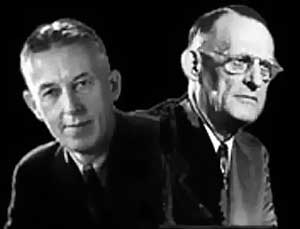This small, black and white vintage photograph shows two men merged into one composite image. On the left, a man with short hair and a smirk wears a sweater over a shirt and tie, with his left side illuminated. His image appears slightly cropped, particularly around his right shoulder. On the right, an older gentleman with slicked-down hair, glasses, and a suit is well-lit on his right side. Both men are seen from the chest up in professional attire, suggesting a business or formal context. The overall quality of the photograph is good, with each man's distinct expression and attire clearly visible.